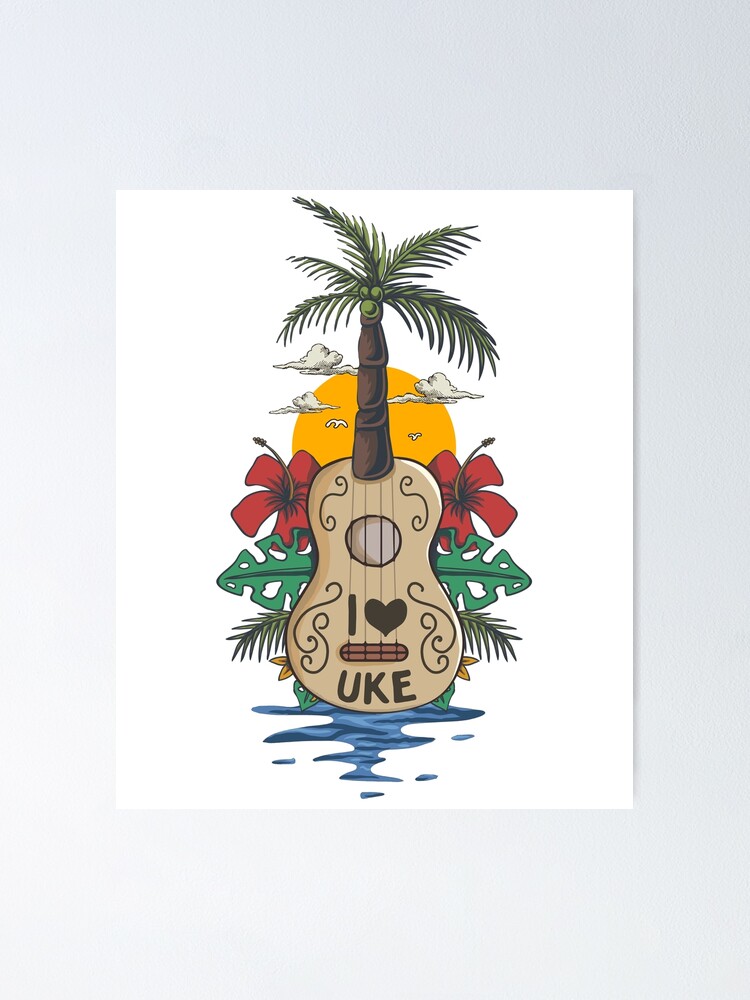The illustration depicts a light brown ukulele standing upright against a white background, framed by a light gray border. The ukulele’s fretboard transforms into the trunk of a palm tree, topped with green leaves and three coconuts. Below the four strings, the body displays "I HEART UKE" in dark nearly black letters, with "I HEART" positioned just above the text "UKE." Embellishing the ukulele are swirly designs on either side. Surrounding the ukulele are red flowers, green monstera and fern leaves, and pine-like leaves extending outward from the waist and lower regions of the instrument. A vibrant yellow-orange sun, accompanied by three small clouds and two white birds, rises behind the ukulele's neck. The scene is completed with whimsical blue water details at the base of the ukulele, forming a shape with droplets around it.